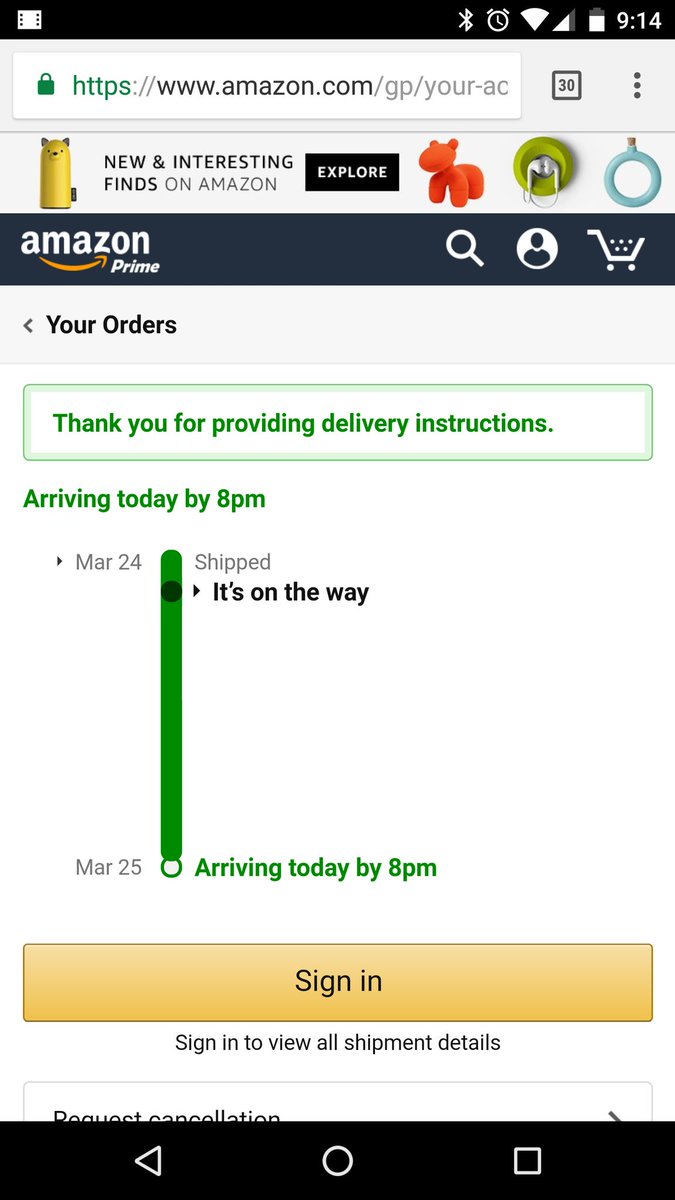A detailed screenshot of the Amazon website, captured on a mobile device such as a tablet or phone. The background is predominantly white. At the very top, there's a slender black notification bar showcasing typical status icons including Bluetooth, an alarm clock, Wi-Fi signal, network signal strength, battery percentage, and the time, which is 9:14. All these icons are aligned to the right-hand side.

Just below the notification bar, there is a search bar with a lock icon indicating a secure HTTPS connection in green lettering followed by the Amazon.com address. Beneath the search bar is a prominent banner displaying "Amazon Prime." On this same banner, to the right, are icons for search, user profile, and a shopping basket.

Further down, the interface displays a section labeled "Your Orders." This is contained within a white rectangle box with the message "Thank you for providing delivery information" written in green letters. It also provides specifics about the delivery timeline, stating "arriving today by 8 p.m." in green letters, and reiterates this information with the date "May 25th, arriving today by 8 p.m." 

Additionally, there is a "Sign In" button for Amazon users and, at the very bottom of the screenshot, the mobile device's navigation bar with buttons for home and back actions can be seen.